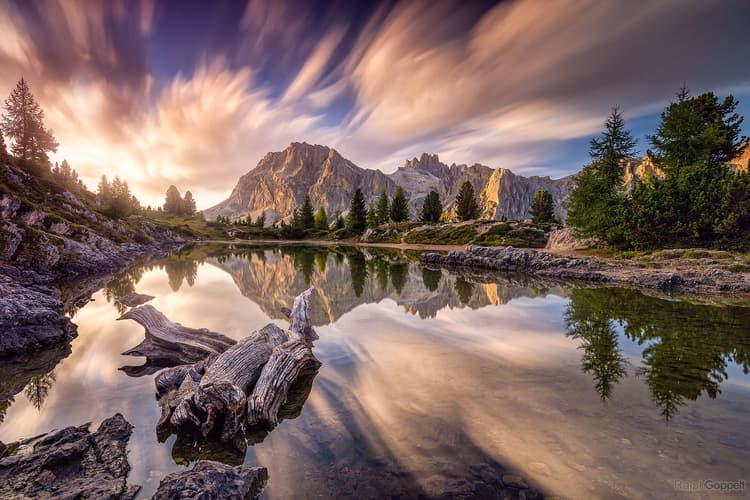This image captures a stunning and serene nature scene that features a breathtaking mountaintop, with its gray peaks suggesting a dusting of snow, reflected perfectly in the calm, clear waters of what appears to be a lake, though it could also resemble a river with no movement. Dominating the scenery is a vibrant, bright blue sky dotted with big, white clouds, some appearing almost hyper-realistic in their starkness and detail. 

Flanking the lake are lush, bright green trees, with some areas casting darker shadows, particularly on the left side of the image where a hill rises. There's a distinct green bush on the right side, also mirrored in the pristine water below. Adding to the natural beauty are elements like a weathered wooden log lying partly submerged in the water and big, giant stones scattered around. The water’s reflective surface captures the dramatic landscape in rich detail, accentuating the picture's artistic quality.

Overall, the scene is one of natural tranquility and stunning visual contrast, offering a snapshot of a bright, beautiful, and calm day in the great outdoors.